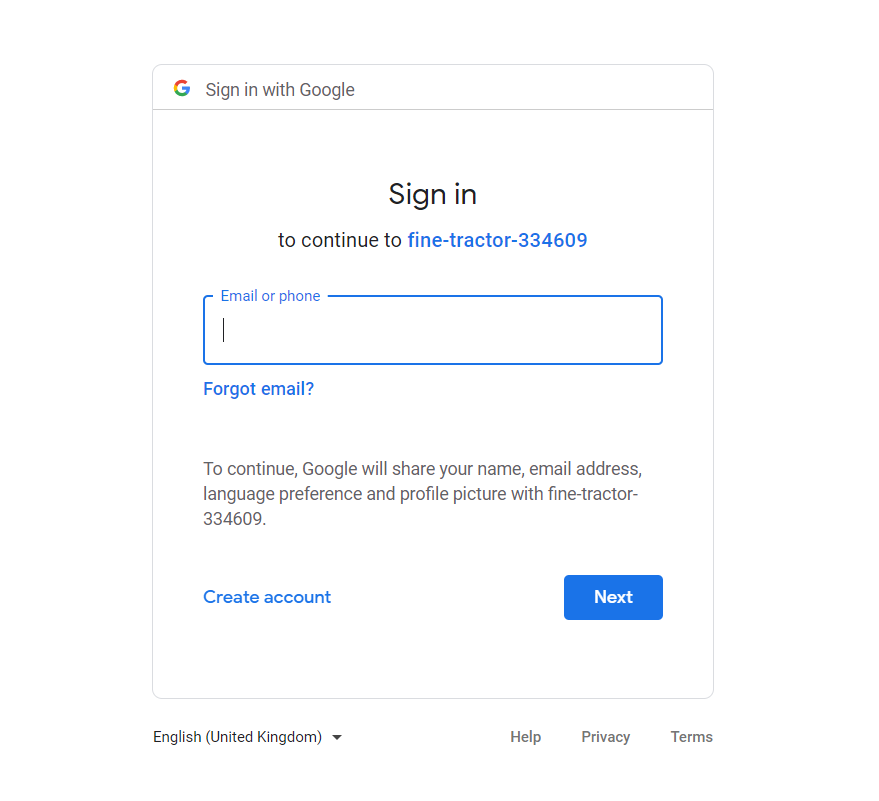This image is a detailed screenshot of a Google sign-in page on a website. At the top of the page, there is a small banner featuring Google's rainbow-colored ‘G’ logo followed by the text "Sign in with Google." Below this banner, in the center of the page, there is a prominent heading that says "Sign in" with a capital 'S.' 

Directly underneath the heading, there is a line of blue text that reads "to continue to findtractor-334609," indicating the service that the sign-in is for.

Beneath this blue text, there is a rectangular input field with a blue border where users are prompted to enter their "Email or phone." Directly below this input field, there is a blue hyperlink that reads "Forgot email."

A paragraph of black text follows, which states: "To continue, Google will share your name, email address, language preference, and profile picture with findtractor-334609." 

Below this informational text, there is another blue hyperlink labeled "Create account." Over to the right side of the page, there is a blue rectangular button with the white text "Next." Outside the button, there is additional text indicating the ability to "Sign out."

At the bottom of the page, there is a small footer. On the left side of this footer, it displays the text "English (United Kingdom)" with a drop-down arrow for language selection. On the right side, it features links labeled "Help," "Privacy," and "Terms."